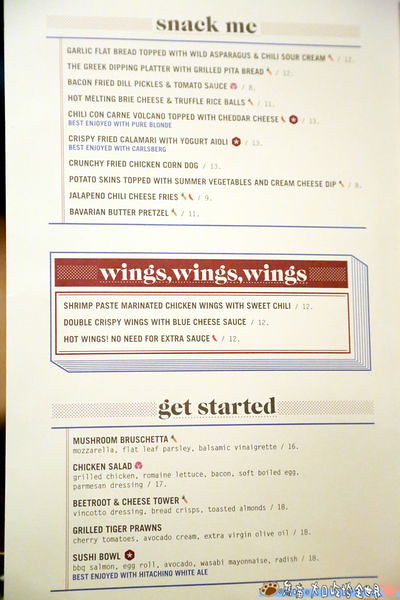The photograph captures a section of a menu, meticulously divided into three distinct categories.

At the pinnacle of the page, under the category title "Snack Me" which is emblazoned in black with a blue underline, an array of tempting snacks is listed. These include:
- Chili Con Carne Volcano topped with Cheddar Cheese
- Crispy Fried Calamari with Yogurt
- Potato Skins
- Greek Dipping Platter
- Garlic Flat Bread topped with Wild Asparagus and Chili Sour Cream
- Bavarian Butter Pretzel

Following this section is another blue line that acts as a separator, leading the viewer's eyes downwards towards the next category centered on the page.

This next section is highlighted by a stylized marquee design. Topping this section is a vibrant red bar with the words "Wings, Wings, Wings" prominently displayed in white text. Within a white rectangle beneath this header, a selection of wing options is showcased:
- Shrimp Paste Marinated Chicken Wing with Sweet Chili
- Double Crispy Wings with Blue Cheese Sauce
- Hot Wings, No Need for Extra Sauce

Finally, at the base of the menu, lies the "Get Started" section, with the category title again marked in black. This portion introduces a variety of starter dishes including:
- Mushroom Bruschetta
- Chicken Salad
- Grilled Tiger Prawns

The thoughtful layout and creative design of the menu ensure a visually appealing presentation that invites patrons to explore the culinary delights on offer.